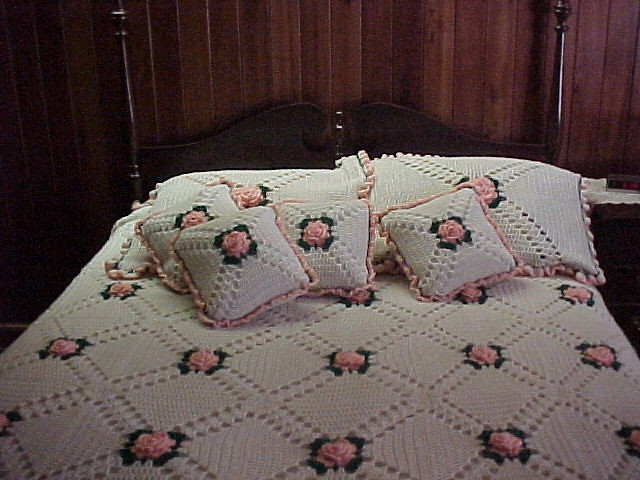This photograph captures a vintage-style bedroom, reminiscent of decor from the 60s or 70s. The image is taken from the foot of the bed, providing a diagonal view down the bed. The back wall is covered with dark, vertically slatted wood paneling, adding a rustic charm to the room. 

In front of this wall stands a large wooden bed frame with distinct architectural features. The headboard has two wooden poles on either side, reaching halfway up the frame. These poles are connected by a gracefully arching wooden piece that starts from the left, curves upward in the center, and then arches down to the right pole, resembling ocean waves meeting.

The bed itself is adorned with a cream-colored, crocheted bedspread that features a pattern of large X's created by interconnected squares. At the junctions where these X's meet, there are intricately sewn pink roses with green leaves. The same design extends to the four small throw pillows and two larger bed pillows placed against the headboard. The pillows share the bedspread's cream base and X pattern, featuring the pink roses prominently in their centers, with the throw pillows also displaying a delicate pink frill around their edges.

This cohesive and charming pattern provides a touch of delicate elegance to the rustic wooden backdrop, creating a harmonious blend of vintage elements and intricate textile craftsmanship.